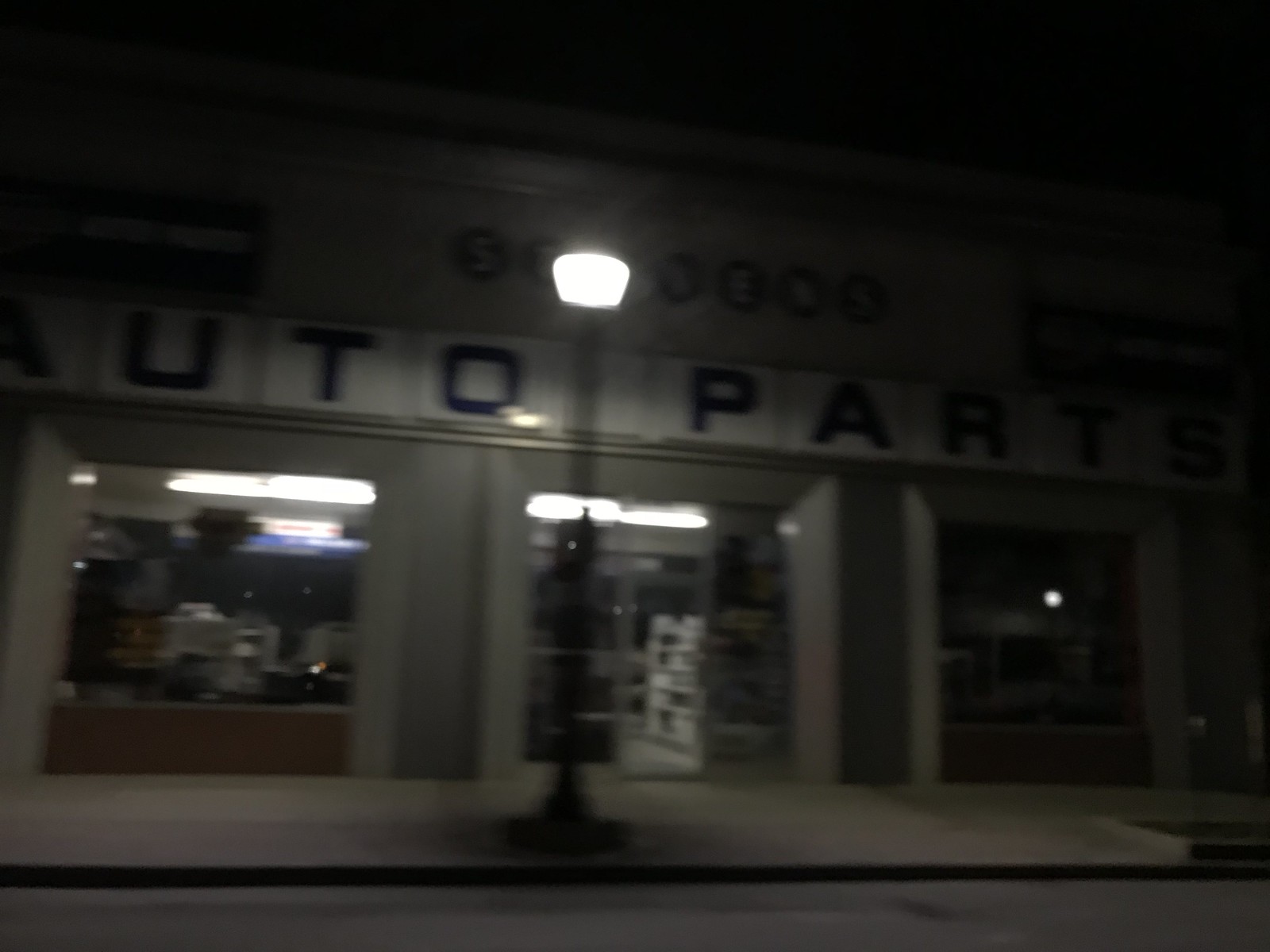This outdoor nighttime photograph, wider than it is tall, captures a blurred view of a city street. Central to the composition, slightly left of center, stands an illuminated lamppost casting a soft glow over the scene. Dominating the background is a storefront with a marquee that reads "Auto Parts." The letters 'A' and 'T' on the marquee are partially obscured by shadows, and additional text above the store is blurred by the lamppost's light. Although the interior lights of the store are on, it seems closed with no visible figures inside. The image's overall fuzziness lends an air of ambiguity, leaving it unclear whether this is a photograph or a computer-rendered depiction of an auto parts store at night.